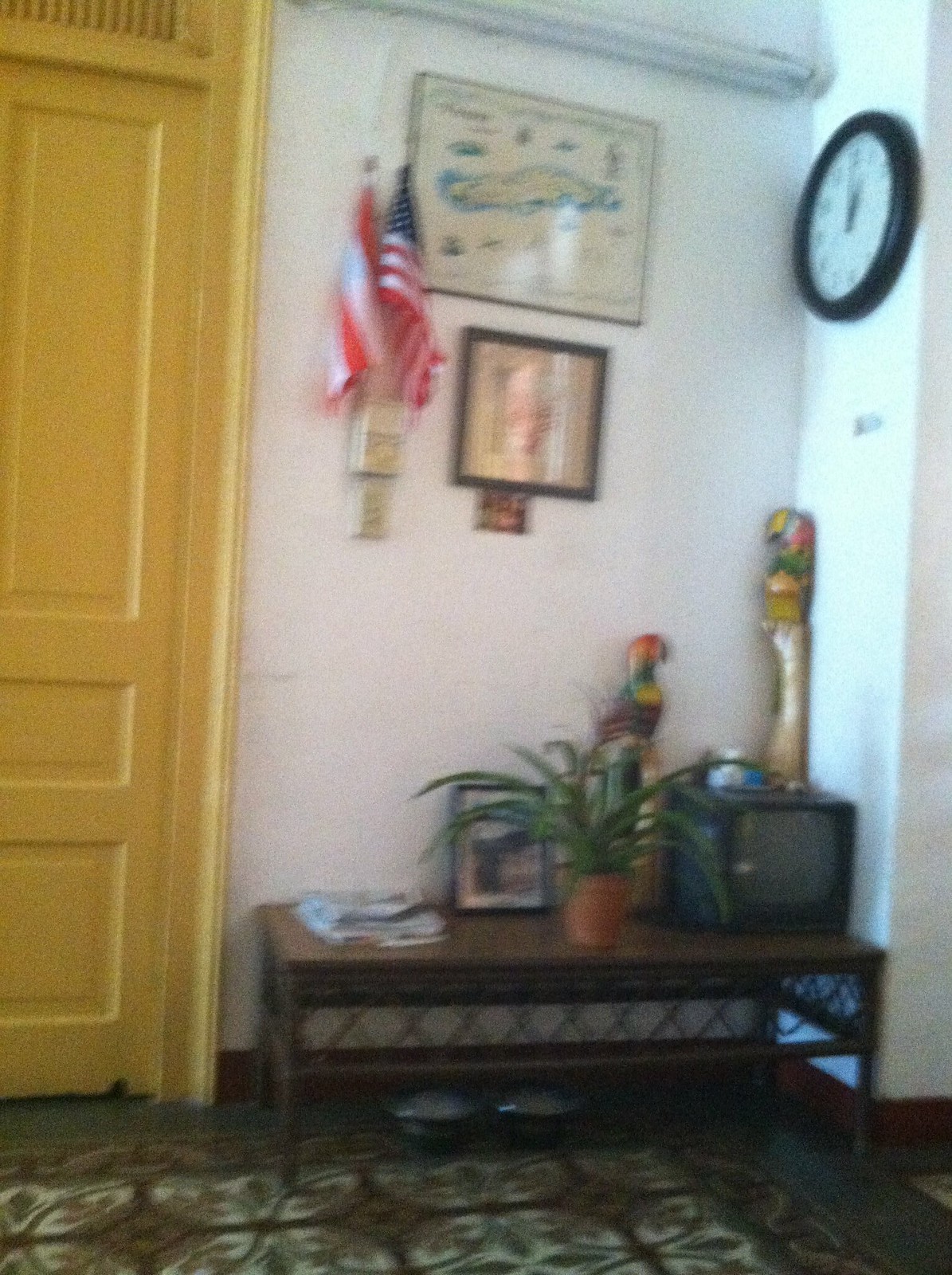This image depicts the interior of a cozy, home-like room, characterized by a mix of traditional and casual decor elements. The room features a pristine white wall, against which a yellow door with a matching door frame stands out. Notably, the door includes an old-fashioned grate at the top, adding a vintage touch.

Mounted parallel to the top of the door is a halogen lamp, providing a warm glow along the white wall. Beneath the lamp, there is a framed picture with a dark border. This artwork appears to depict a light-colored landscape surrounded by water, all set against a white background. The picture is adorned with black lettering and a few small icons that are difficult to discern.

Below this picture is another framed image, also with a dark frame, but its details are not easily distinguishable. To the left of the artwork, two flags are displayed: an American flag and another red and white flag of unspecified origin.

Additional elements in the room include a small, cube-shaped, old-style television with a thicker back, typical of older models. This TV is accompanied by various knickknacks and a potted plant, adding a touch of personality and greenery to the space. Overall, the room exudes a charming blend of nostalgia and homeliness.